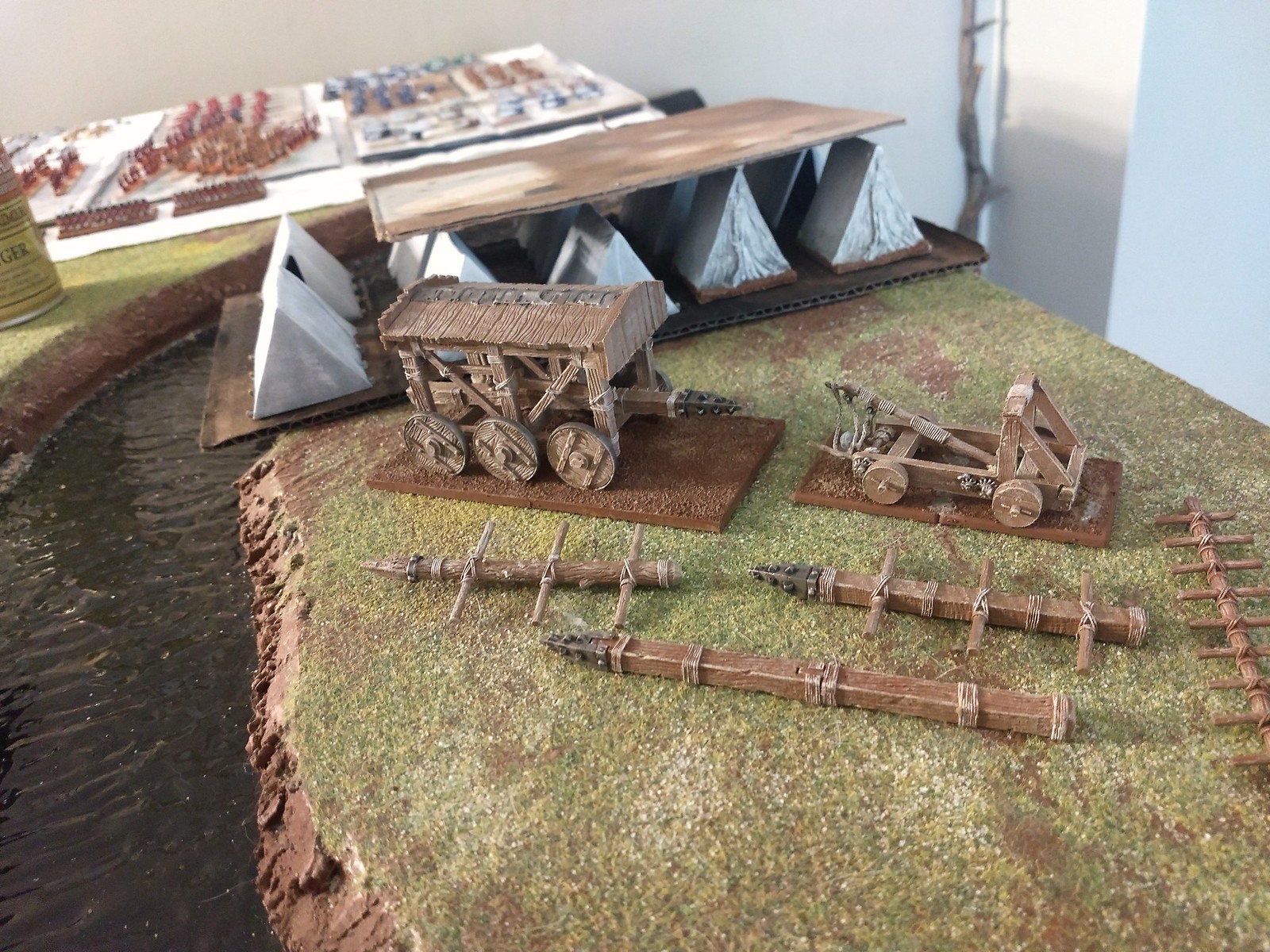The image depicts a meticulously crafted scale model of an ancient campsite. Centered towards the upper part of the model, there are eight white teepees arranged in a row between two pieces of cardboard. Below this, slightly to the left, is a detailed wooden carriage, while a cart is positioned to its right. Near the bottom-center, spears are laid out on a patch of green fake grass. To the left of this grassy area, a blue river bends around the central piece of land, creating a moat-like feature.

Adjacent to the grassy patch are medieval implements of war, including a wooden catapult, a battering ram, various ancient ladders, and a trailer with six wheels. Scattered brown dirt and clay figures enhance the rustic feel of the scene, depicting the aftermath of an ancient battle. Tiny figurines of men, colored in blue and red, are positioned behind the tents, capturing the sense of a battleground. The whole model rests on a base that mimics natural terrain with green grass and brown dirt, giving it an authentic look. In the background, the actual room with white walls is visible, emphasizing that this is a hobby creation, likely representing a historical campsite or battleground.